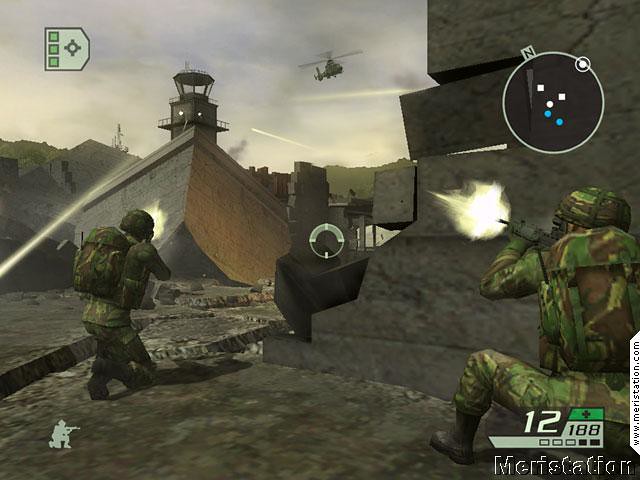The screenshot captures an intense moment from a video game featuring two soldiers in camo gear engaged in a firefight. Both soldiers are kneeling on one knee, aiming and firing their weapons, with visible yellow muzzle flashes emanating from their guns. The soldier on the right is positioned slightly ahead of his comrade, and directly above him, there is a circular mini-map displayed, which features white and blue dots against a black background, indicating various points of interest or enemy positions.

In the foreground, scattered gray rocks offer minimal cover for the soldiers. Dominating the middle of the image, a helicopter hovers in the air, enhancing the combat scenario's dynamic nature. Behind the helicopter, a large, gray-colored tower can be seen, which appears to be part of a crashed ship.

Amid this grayscale environment, a white circular crosshair is centered in the image, potentially indicating a targeting or aiming system. In the top left-hand corner, a nearly square-shaped UI element displays a mix of black, green, and white icons, including a small white soldier icon.

Toward the bottom left and right corners, various interface elements are visible. The bottom right corner features lettering, likely part of the game's HUD, displaying the word "Mary Station" or a similar term. Above this lettering, the ammunition count is shown: '12' in white text followed by '188' in black with a gray background. A small green square sits above the ammo counter, while two additional squares below the '188' are also present, one white and the other black, possibly indicating other resources or gameplay statistics.

The overall scene is meticulously detailed and indicative of a tactical and immersive gaming experience.